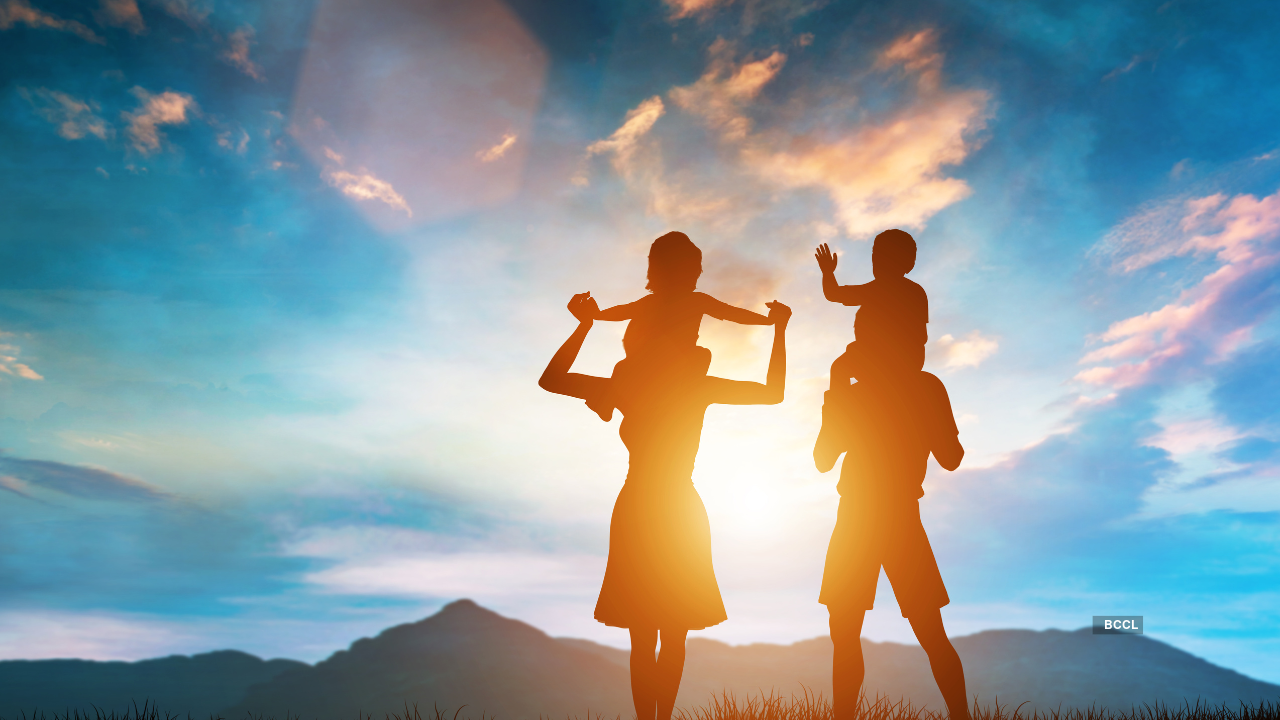In this evocative photograph, we see the silhouetted profiles of a family of four—two adults and two children—against a vivid sunset. On the right side, the dad stands tall in shorts, holding a young boy on his shoulders. The boy raises his left arm in a friendly wave. To the left, the mom, dressed in a skirt or dress, carries a young girl on her shoulders. She holds the child's hands securely. The setting sun casts a warm, whitish-yellow glow, painting the sky in shades of blue with hints of yellow-pink and even purplish-red. The sun's reflection gleams through the clouds and peeks between the parents at their feet, casting an almost octagonal shimmer. At the base of the image, there's a faint silhouette of hills and mountains, with patches of grass visible, grounding this touching family scene in nature.